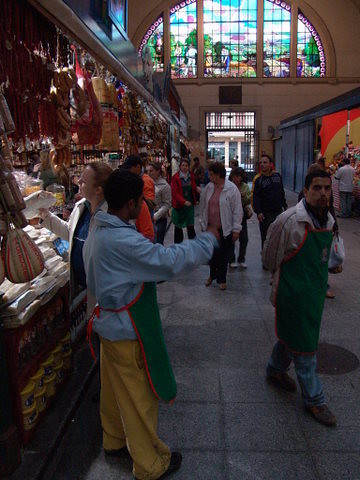The image captures a bustling indoor market scene with a variety of kiosks and pavilions selling handmade items. To the left, numerous handcrafted handbags are displayed prominently. In the foreground, a gentleman dressed in yellow pants, a blue shirt, and a green apron with red trim is waving at another man who is wearing a green apron over a white collared shirt, blue jeans, and brown shoes. These men appear to be vendors engaging with the busy crowd around them. To the right, several individuals are gathered near another pavilion area, with some people donning pink, white, and red shirts. In the background, there is a large square door that allows natural light to filter in, and above it, a grand stained-glass window is visible. This window depicts scenes possibly involving people in a field with green trees, contributing to the festive or religious ambiance. The stone-tiled ground further accentuates the historical or rustic feel of the market.